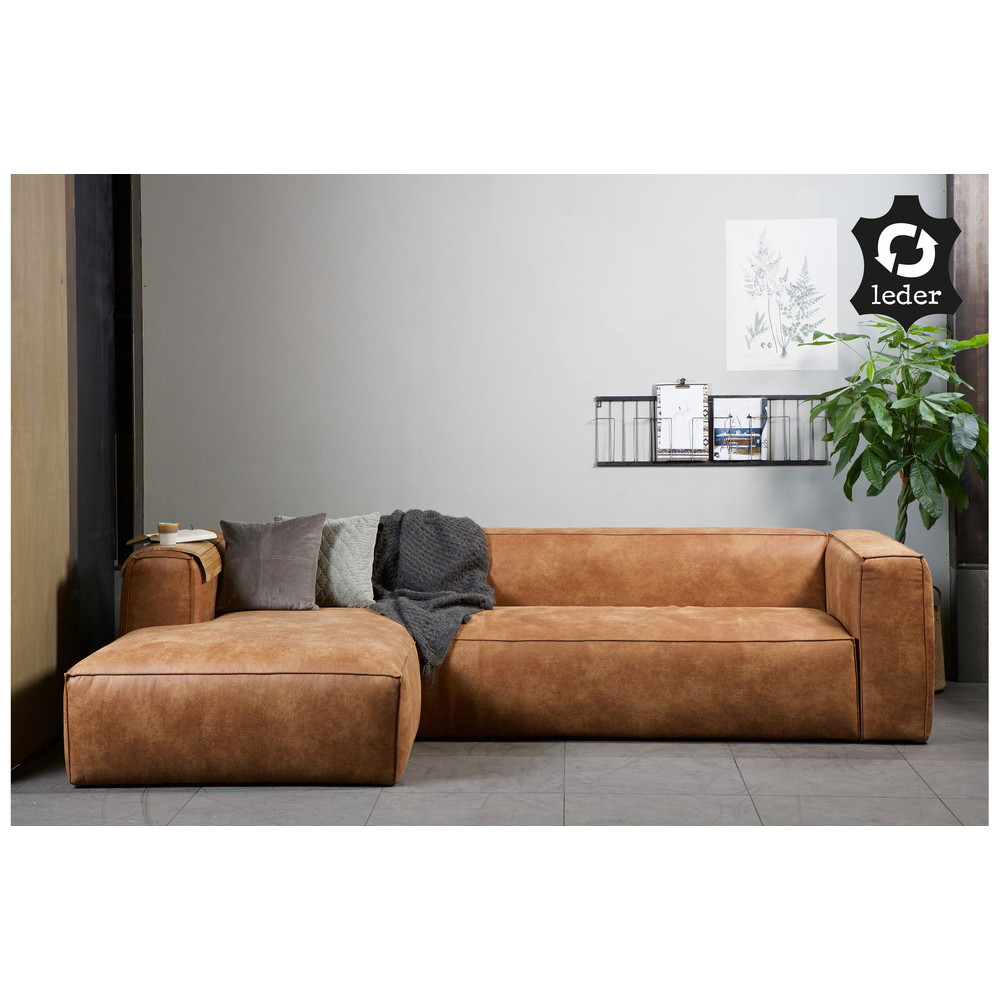This image showcases a light brown sectional sofa positioned lengthwise against a white tile or marble floor, giving the room a sleek, clean look. The sofa, resembling the color of saddle leather, backs up to a wall and features a chaise lounge protruding from its left end. On the left corner of the sofa lie two throw pillows alongside a gray blanket. A mysterious object rests on the arm of the sofa at the far left. Directly behind the sofa, a wall-mounted holder stashes magazines and similar items, while above it hangs a picture poster depicting a small tree. In the right corner behind the sofa, a tree-like plant adds a touch of green to the room. Elevated above this plant, a black sign sporting a recycling symbol and the text "LEDER" stands out. The setting, characterized by its light hues and professional ambiance, suggests it could be a business environment, much like a doctor's office.